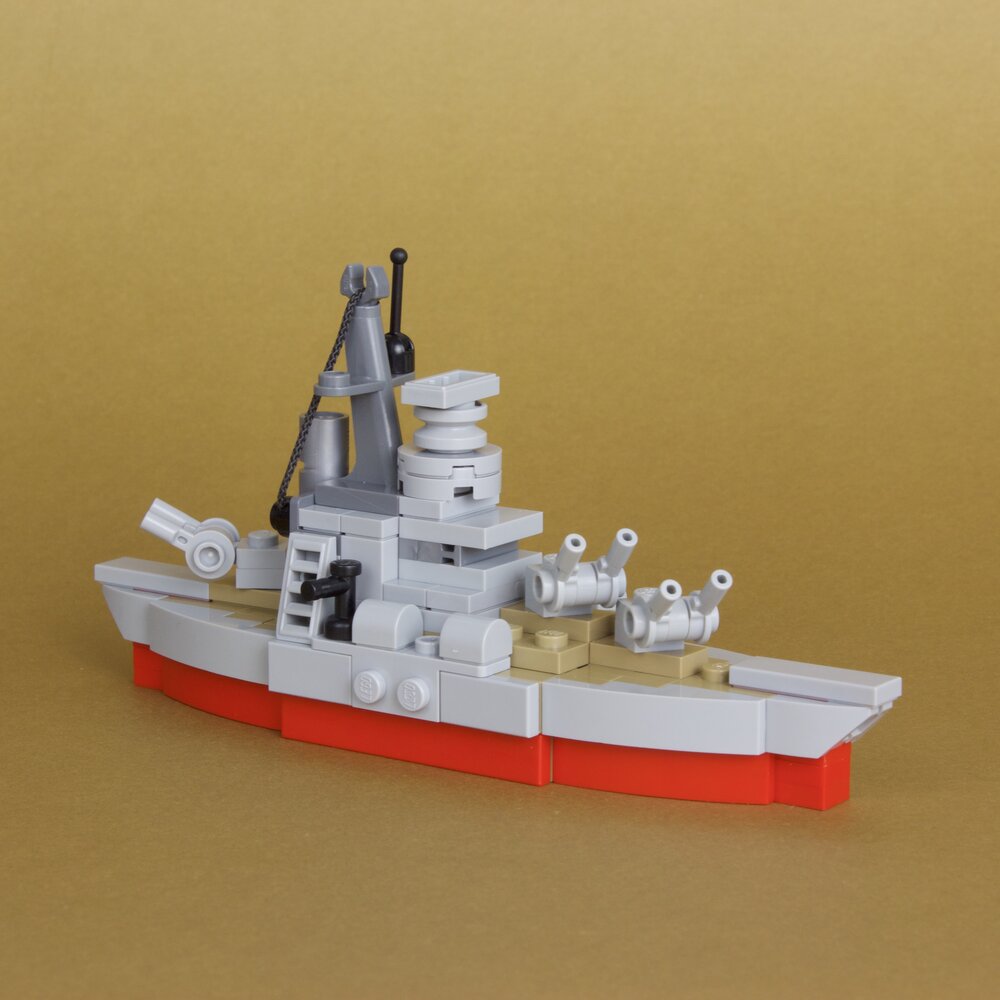A realistic photograph depicts a small Lego-style PT boat displayed against a tan background, resembling the interior of a shoebox. The boat features a bright red bottom layer, followed by gray sides, and a deck crafted from white and beige Lego blocks. On the left side of the boat, a large double-barreled gun is pointed upwards towards the sky. The boat's complex superstructure includes a white ladder leading to the top of the captain's house, which supports two gray smokestacks connected by a cable to the area where another double-barreled gun is oriented towards the rear of the boat. The front of the boat is equipped with two additional double-barreled guns, also pointed skyward. Additional details include a radar, a mast, an antenna, and what appears to be a crane, all constructed from various shades of gray Lego pieces. The meticulous design closely mimics a Navy gunboat, complete with a realistic array of weaponry and equipment, all intricately assembled from Lego-style blocks.